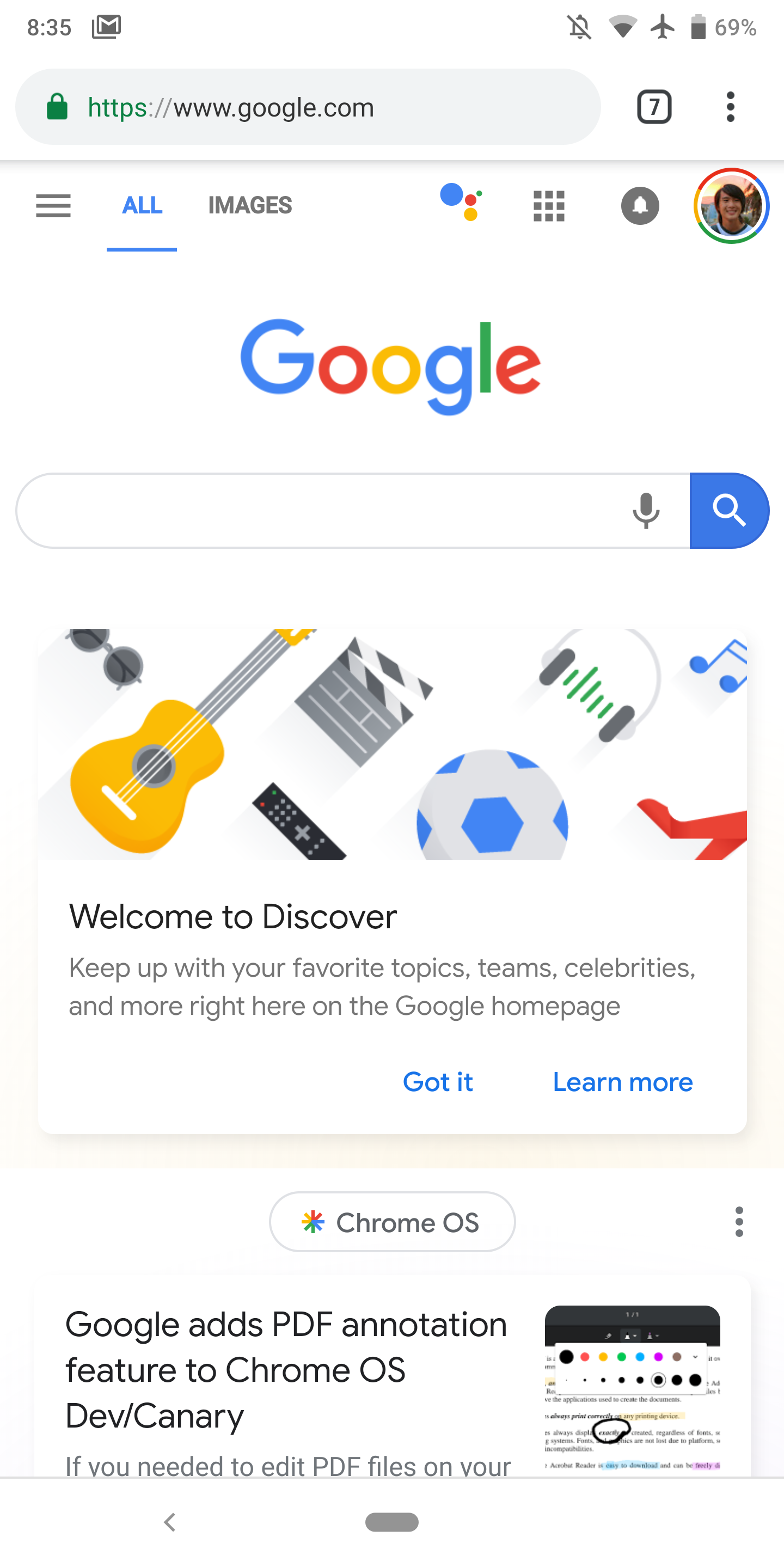The image is a screen capture taken from a digital device, displaying the Google homepage. The top of the screen features the URL, written in green and black text, as "https://www.google.com." The background of the page is predominately white, enhancing the cleanliness and simplicity of the design.

Centered on the page, we find the prominent Google logo, composed of vibrant letters in blue, red, yellow, blue, green, and red. Directly below the logo is the well-known Google search bar, inviting users to enter their queries. Above the logo, positioned just below the address bar, are clickable options, including “All”, highlighted in blue, and “Images,” indicating available search categories.

In the upper right corner of the screen, there is a circular profile photo, likely representing the current user logged into the account. Scattered below the search bar are various colorful icons: starting from the left, an image of sunglasses, a yellow guitar, a white and blue soccer ball, and on the far right, a red high-heeled shoe. These icons add a touch of vibrancy and visual interest to the otherwise minimalistic page design.